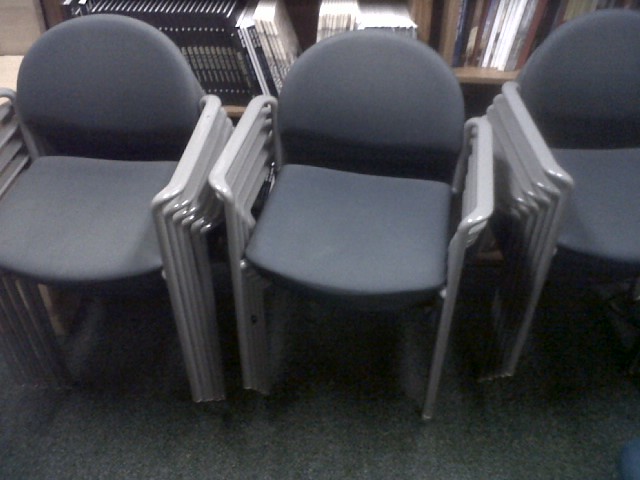The image depicts a typical office setting featuring three stacks of chairs, each stack containing five or six chairs. The chairs are designed with navy blue cushioned seats and backrests, complemented by yellow armrests and framed in a silver-gray metal or plastic. These chairs are placed in front of a wooden bookcase filled with an assortment of books. Some books are arranged in uniform groups, with about 30 identical ones and another set of similar white books, while others are more varied in appearance. The room's flooring is covered with dark blue or gray office carpet tiles, enhancing the professional atmosphere and matching the color scheme of the chairs.